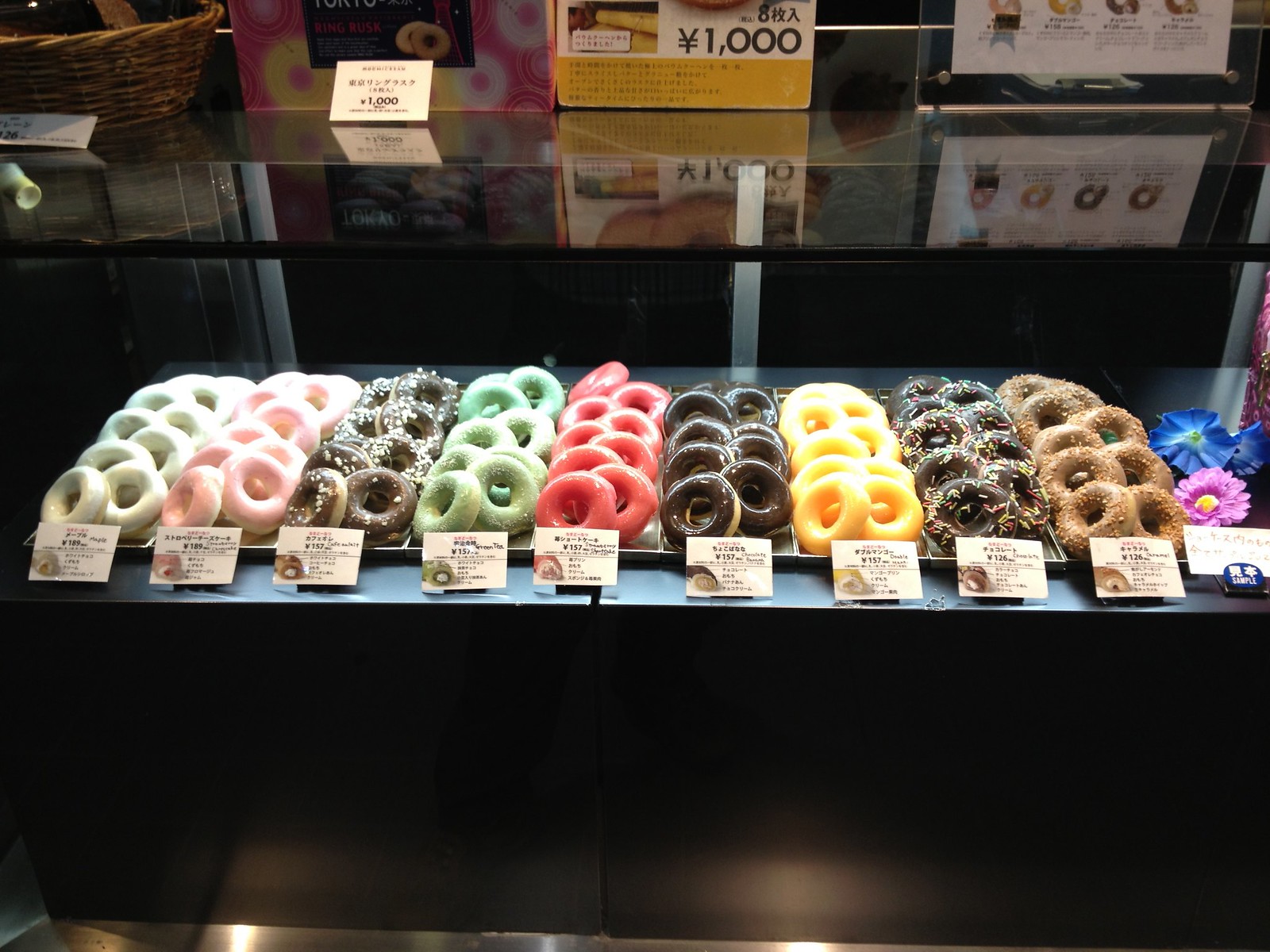This photograph showcases a display cabinet in a bakery, likely located in Asia, featuring an array of vibrant, multi-flavored donuts. The cabinet, which is made of glass and has a solid black frame, contains ten meticulously arranged trays of rectangular donuts, each boasting different glazes. Starting from the top, one can see white-glazed donuts, followed by ones with pink glaze, chocolate donuts adorned with colorful sprinkles, and green-glazed donuts. Other trays include bright pink-glazed donuts, plain chocolate-glazed donuts, regular clear-glazed donuts, chocolate donuts with long colorful sprinkles, and a unique coffee-colored glaze topped with nuts. On top of the glass cabinet, several boxes prominently display pricing in yen, highlighting its Asian location. Despite the darkness of the overall image, strategic lighting ensures the donuts are the focal point, with detailed display tags written in Chinese in front of each variety further emphasizing their distinct options.